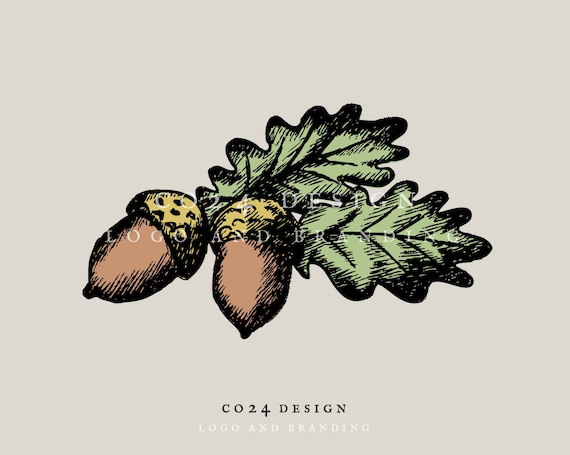The illustration features two centrally positioned acorns against a stone-colored, beige background. The acorn on the left is light brown with a mustard yellow to brown cap, detailed with black dots and an etched black shadow outline. The acorn on the right, similar in coloration, is oriented with its point downward. Both acorns sprout sand green leaves, marked with black vein outlines. Overlaid text reads "CO24 Design" in black with "Logo and Branding" in white beneath it, and the same text appears as a white watermark over the acorns. The overall image resembles a sketch, characterized by its detailed line work and illustrative style.